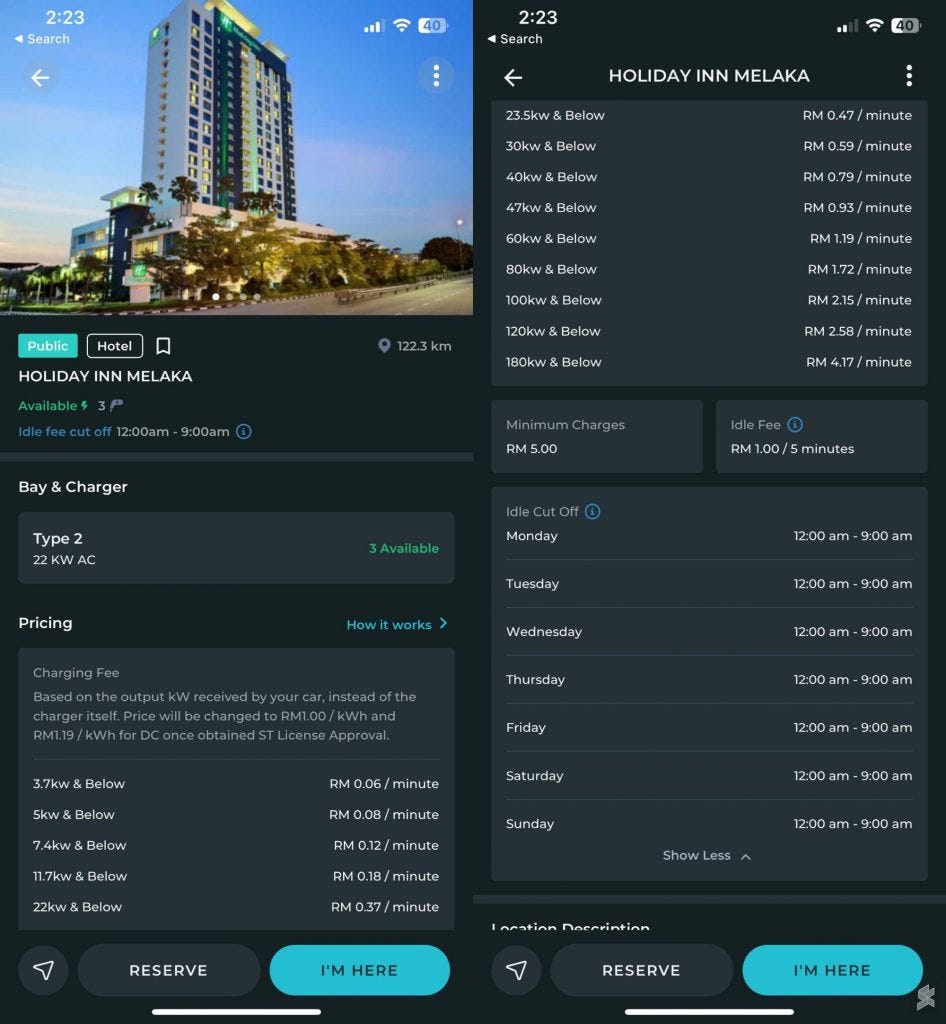The image appears to be a detailed screenshot from a computer screen displaying information about the Holiday Inn Malacca, possibly related to its electric vehicle charging facilities. In the upper left corner of the screenshot, there is a picture of the hotel, portraying it as a tall structure slightly elevated on a hill, surrounded by trees and set against a clear blue sky.

Above the hotel's name, "Holiday Inn Malacca," there is a blue-highlighted text reading "public," indicating the availability status of the charging station. The section underneath also confirms "available" status. The right side of the image displays various informative boxes. One of these boxes shows details about the charging bays and types available, specifying "Type 2, 3 available."

The pricing section elaborates on the charging fees, which are based on the kilowatt output received by the car rather than the charger itself. For example, on the left side, it mentions 80 kilowatts with a rate of RM 1.72 per minute. Further down, there are details about the idle cutoff times, listing specific times for different days, such as Monday and Tuesday from 12 am to 9 am.

At the bottom of the image, there is a button labeled "I'm here," which seems to be clicked, possibly indicating that the user is confirming their presence to use the charging station. The comprehensive details suggest that the facility is meant for hotel visitors to charge their electric vehicles conveniently.